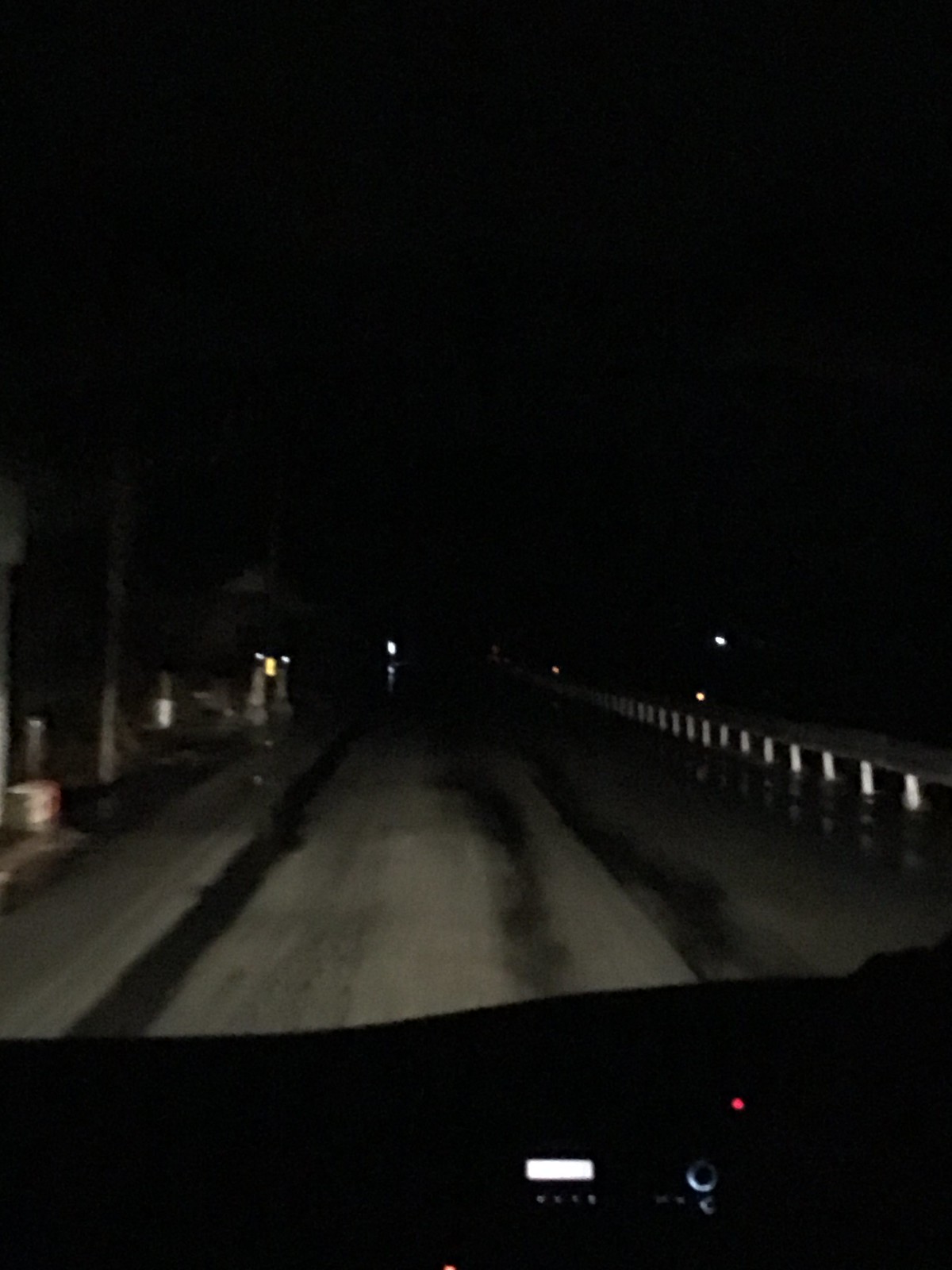A nighttime photograph captures the view from inside a moving vehicle, looking through the windshield as it traverses a bridge. The interior of the vehicle reveals colorful dashboard controls, contrasting with the predominantly dark, grayscale scene outside. To the right, a railing lines the edge of the bridge, offering glimpses of the void below. On the left, a barely discernible structure, possibly a small building or a toll station, stands hinting at its purpose, though the image's blurriness makes it difficult to identify with certainty. Distant lights punctuate the horizon, suggesting a sparse presence of other vehicles or infrastructure far ahead. The solitary vehicle appears to be the only one on this stretch of the roadway, emphasizing a sense of isolation and the quiet stillness of the night.